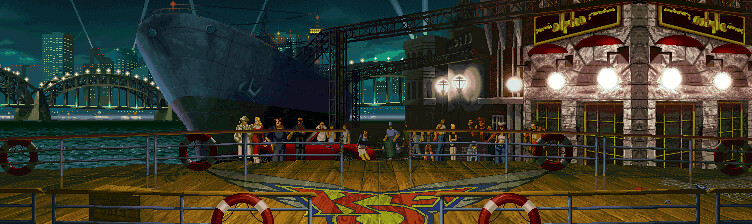This vibrant drawing combines elements of both painting and sketching to create a vivid nighttime cityscape. The artwork features a long, slender, horizontal rectangle that captures a bustling urban scene.

On the left side of the image, a deep, dark blue sky sets a nighttime atmosphere, underlined by a series of high-rise buildings that loom in the distance, also shaded in dark blue. Strikingly lit against the night sky is a gray bridge adorned with arches, each crowned with little white lights that pierce through the darkness. 

Beneath the bridge, the city continues to shimmer with scattered lights, reflecting off a body of water whose type is indistinguishable in the somber light. Dominating the left portion of the scene, a massive ship is docked, its presence emphasized by the adjacent metal scaffolding. The topmost part of the scaffolding serves as a walkway, leading via a probable ramp or ladder into the ship, although no figures are visible. 

Transitioning to the middle and right side of the image, a substantial stone building comes into view, standing prominently on a corner. The building appears to bear the word "ALPHA" in elusive gold letters. This edifice is characterized by four large windows, each segmented into twelve yellow panes. Below the ambiguous signage, four arched red canopies provide a striking contrast, while bright white lights envelop the structure, highlighting its significance in the scene.

Occupying the deck in the foreground are numerous people, likely passengers waiting to embark. The wooden deck shows further signs of maritime life, like railings adorned with life preservers. In the midst of this detailed foreground, a large, winged emblem is painted on the floor, adding an intriguing yet cryptic layer to the scene.

Overall, this meticulously detailed piece captures the essence and dynamism of city life by night, blending architectural grandeur with nautical elements.